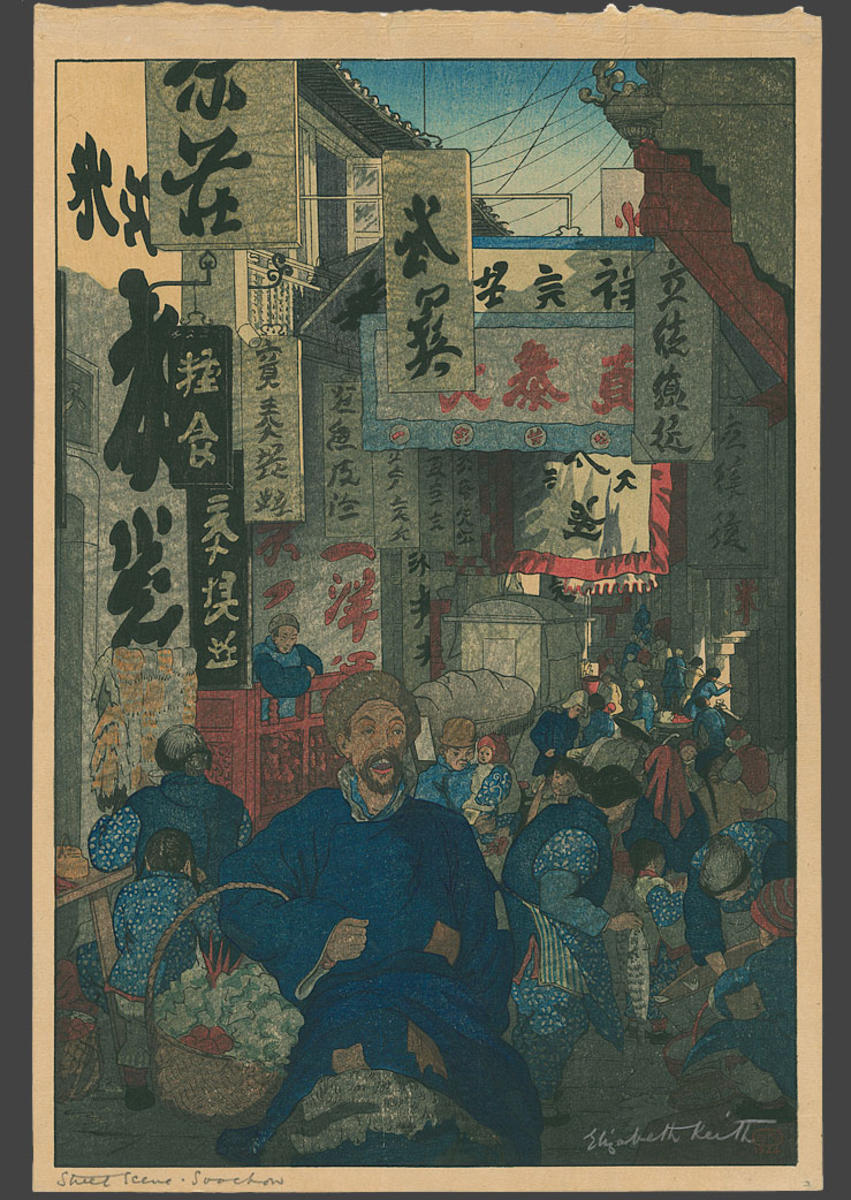The illustration is an intricate ukiyo-e Japanese print depicting a bustling market street under a bright, blue sky. The vivid scene is alive with numerous people engaged in various activities, such as bartering, buying food, and fish, amidst rows of open-air market stalls. The crowd is predominantly dressed in blue and red garments, infusing the artwork with a harmonious palette of blue, red, and grey. Numerous banners and signs, adorned with unfamiliar Asian lettering, hang from walls and balconies, contributing to the market's vibrant and authentic atmosphere.

An interesting focal point is a contented man in a blue cloak, holding baskets as he exits the market, signifying the end of a successful shopping trip. To his left, a vendor's shop brims with Asian prints, each adding further detail to the lively scene. Above, black lines reminiscent of telephone or electrical wires stretch across, enhancing the feeling of a typical, bustling day. 

The print features the artist's distinctive marks: a signature in the bottom left corner and another inscribed in off-white over the artwork at the bottom right. The entire composition, framed within a visible outer border, hints at the artist's meticulous attention to detail and the traditional printmaking techniques employed in its creation.